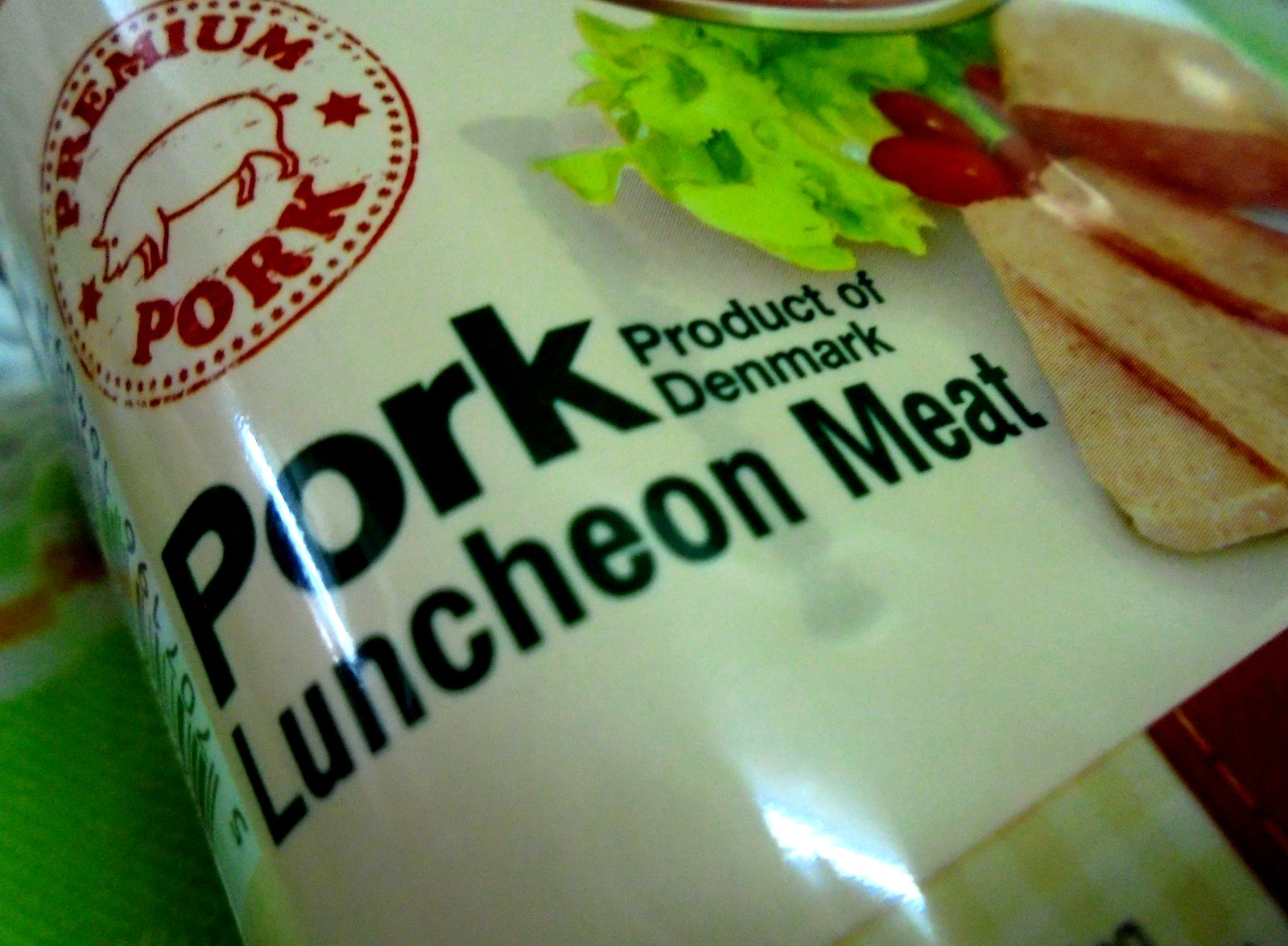The image showcases a packaged food item wrapped in plastic, featuring a striking design. Dominating the top of the package is a red circular logo that frames a drawing of a pig. Above the pig, bold red letters spell out "PREMIUM," and below it, the word "PORK" is displayed. Flanking the words are two six-sided stars. Just beneath this logo, large black lettering declares "PORK LUNCHEON MEAT," also noting that it is a product of Denmark. To the right side of the packaging, a photograph vividly depicts fresh greens, including a vibrant green piece of lettuce, a pair of bright red cherry tomatoes, and several light brown slices of bread. The entire package rests on a green cloth adorned with a white and red pattern. The glossy surface of the plastic wrap catches the light, adding a reflective sheen to the presentation.